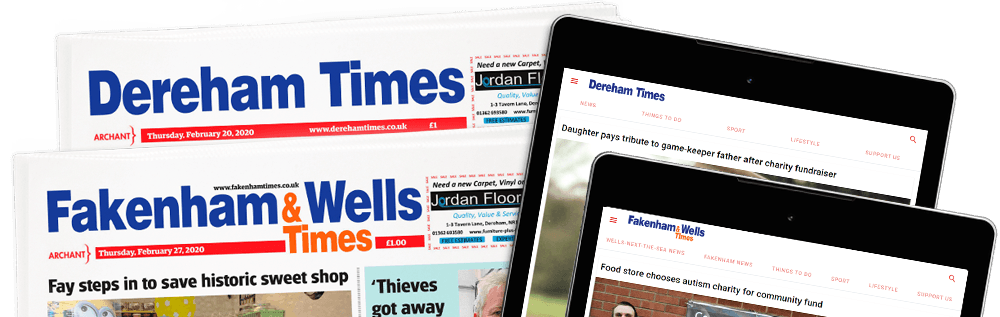In this image, we see an announcement for the digital adaptation of two newspapers. On the left-hand side, two printed newspaper editions are displayed. The top newspaper is “Dereham Times” (D-E-R-E-H-A-M Times), and below it is the “Fakenham & Wells Times” (F-A-K-E-N-H-A-M & Wells Times). Both newspapers feature bold headlines printed on white paper and carry an advertisement for Jordan Flooring on the right side. A red banner beneath each newspaper states the publication dates: "Archant Thursday, February 27, 2020" for the Dereham Times, and "Archant Thursday, February 20, 2020" for the Fakenham & Wells Times.

To the right of the printed newspapers, two digital tablets are shown. Each tablet mirrors the newspapers’ front pages. The tablet on top displays the “Dereham Times” with the headline, "Daughter Pays Tribute to Gamekeeper Father After Charity Fundraiser." The tablet below it features the “Fakenham & Wells Times” with the headline, "Food Store Chooses Autism Charity for Community Fund." Both tablets have a sleek black border, emphasizing the modern transition of these traditional newspapers into digital format.